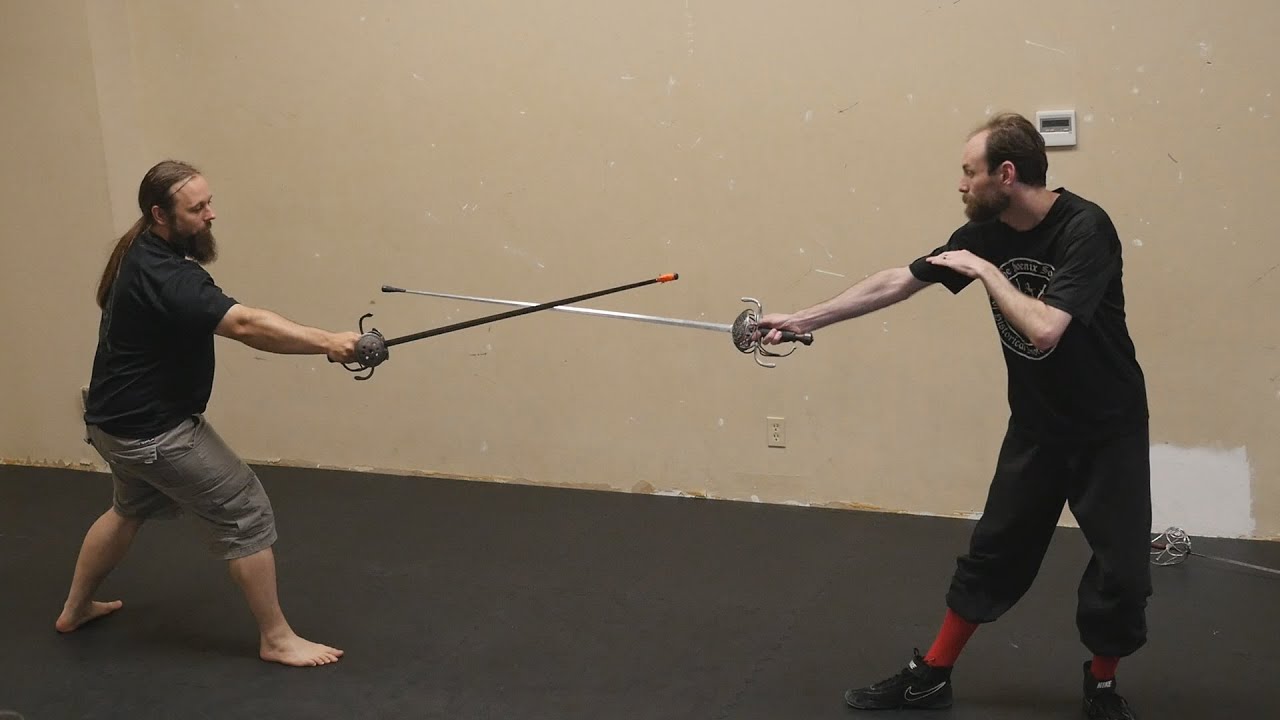This image captures an intense moment of a fencing match between two men. On the left, a long-haired, bearded gentleman in a black t-shirt and gray shorts stands barefoot in a classic on-guard stance, his rear foot perpendicular to his forward foot. Meanwhile, his opponent on the right, dressed in a black t-shirt, baggy black pants, red socks, and black running shoes, mirrors his stance. Both are equipped with foils or possibly épées, distinguished by their small, circular hand guards adorned with curvy embellishments. Against a backdrop of a light brown wall marred by white nicks, possibly from previous fencing encounters, they hold their swords crossed, poised for action. The dark beige wall and the contrasting black floor emphasize the scene's dramatic tension, accentuated by a solitary extra sword lying in the bottom right corner. The man on the right also makes a distinctive gesture with his left hand, palm down towards the ground. This image clearly depicts the ready phase of their fencing bout, highlighting the anticipation and precision characteristic of the sport.